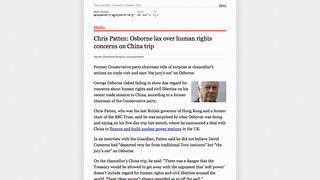The image depicts a distant shot of a piece of text, making the details somewhat challenging to decipher. The content consists of extremely small black text. A key focus is the word "media," highlighted in red, with a long red underline beneath it. Following this, there is another segment of black text that includes the phrase "crisp pattern" alongside two small dots. The text appears to reference a person named Osborne in the context of raising human rights concerns during a trip to China. Below this segment, the text continues with approximately four paragraphs of information, all in very small black font.

Among the body of text, one sentence is distinctly set apart in blue, both in color and by an underline. Additionally, the image includes a photograph of an elderly man, who appears to be in his early to late 70s with white hair, enclosed in a gray square.

The overall layout of this informational area is flanked by two vertical light gray rectangles, one on the left and one on the right, framing the central content symmetrically.